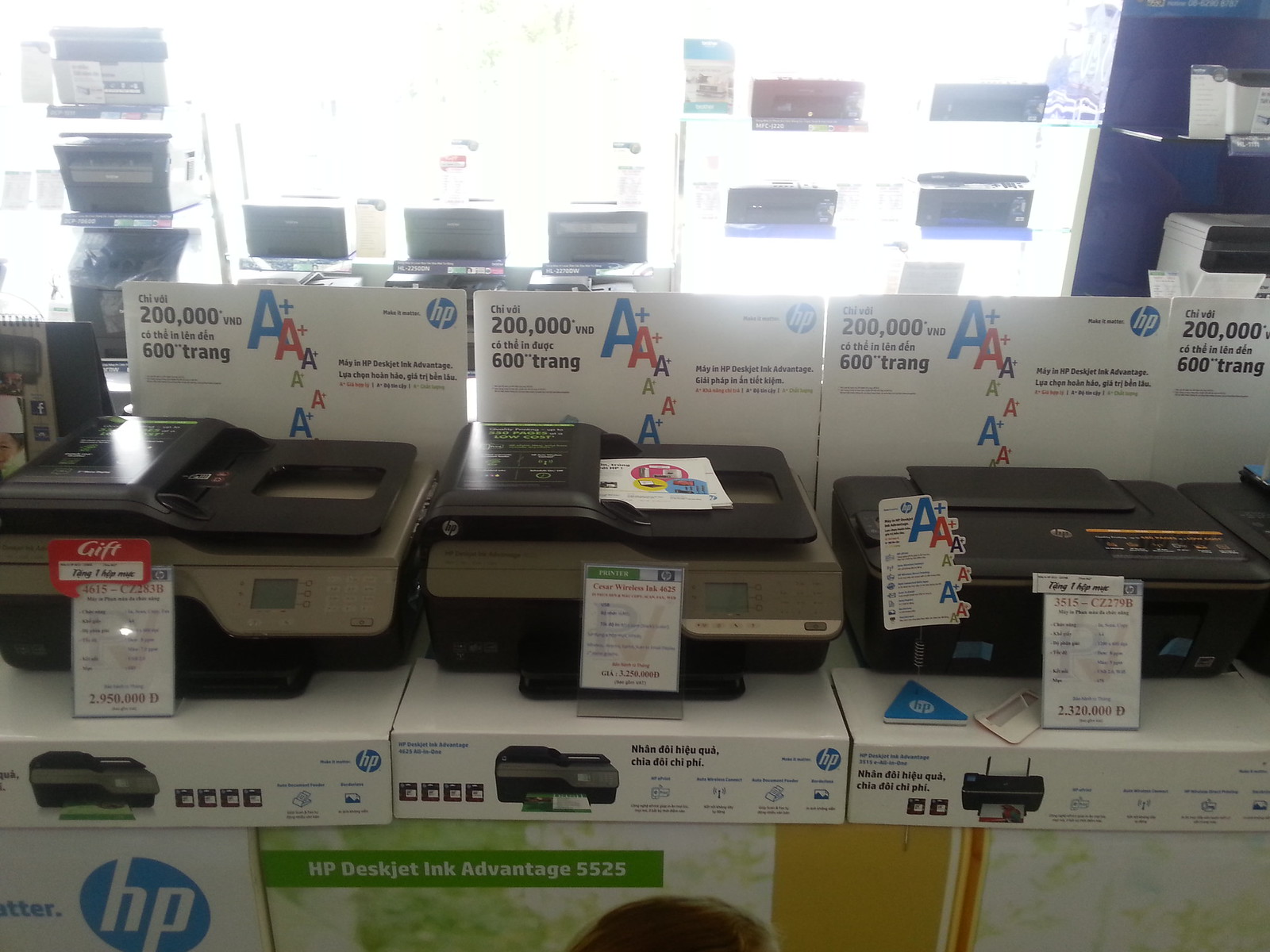This photograph features a display of three black HP DeskJet Ink Advantage 5525 printers prominently placed on a white platform in a Vietnamese store, evident from the language on the signage. Each printer, showcasing inbuilt scanners, is resting on boxes marked with the HP logo— a blue circle with white "HP" text. Below the printers, a blue banner clearly states "HP DeskJet Ink Advantage 5525." The background reveals more printers on shelves against a glass window, with sunlight streaming through, causing a slight overexposure in that part of the image.